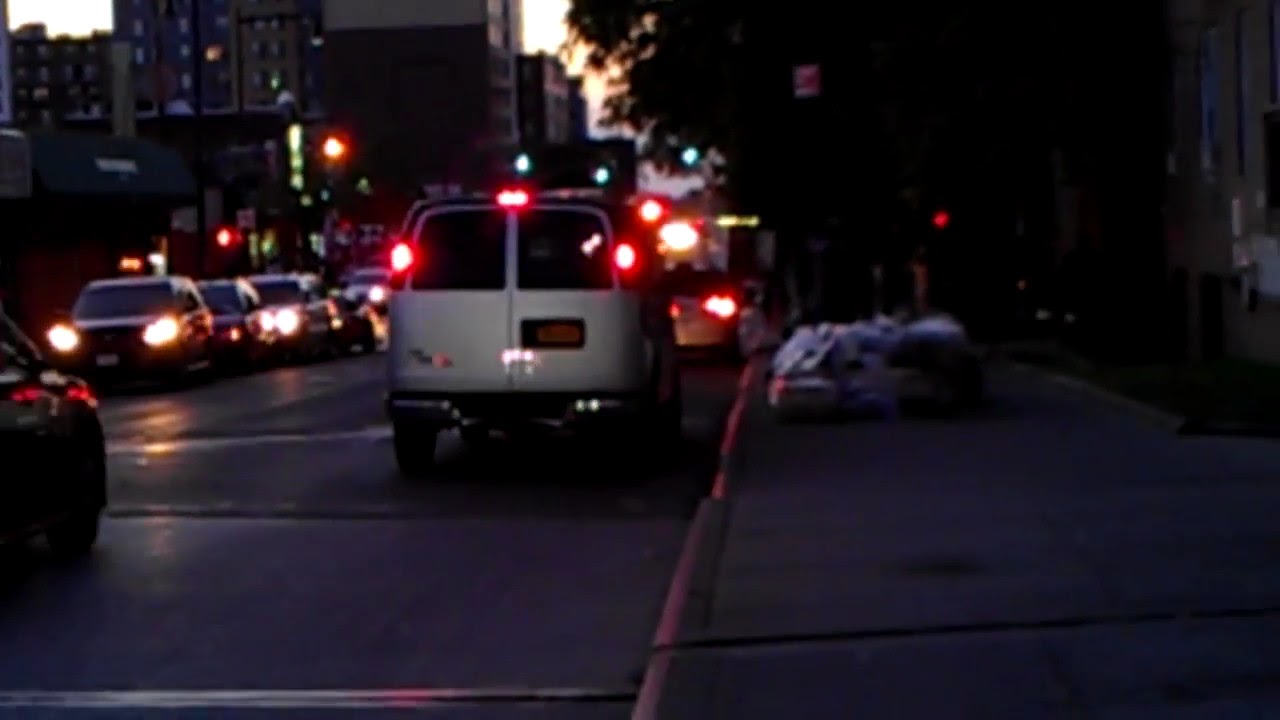The image depicts a busy urban street scene, likely in the early morning or late evening, as suggested by the dim, transitioning light. In the foreground on the bottom right, there is a sidewalk while the bottom left shows a street bustling with cars, their headlights and brake lights creating scattered points of bright light against the city's dusk. The closest object to the center is a white van facing away, its red brake lights glowing prominently. To the left of the van, a row of approximately four or five cars lines the street, each with their headlights on. Traffic lights are visible, with one showing green and another red, signaling the bustling flow of vehicles. In the top left corner, several buildings, potentially offices or apartments, stand with their small rectangular windows faintly visible. The top right features a large tree, and a sliver of the sky peeks through the center of the image. The color palette ranges from white, black, and gray to red, yellow, green, and tan, adding to the picture's vibrant yet subdued city atmosphere. The image provides a ground-level perspective as if taken by someone standing on the sidewalk, capturing the essence of a busy urban environment at twilight.